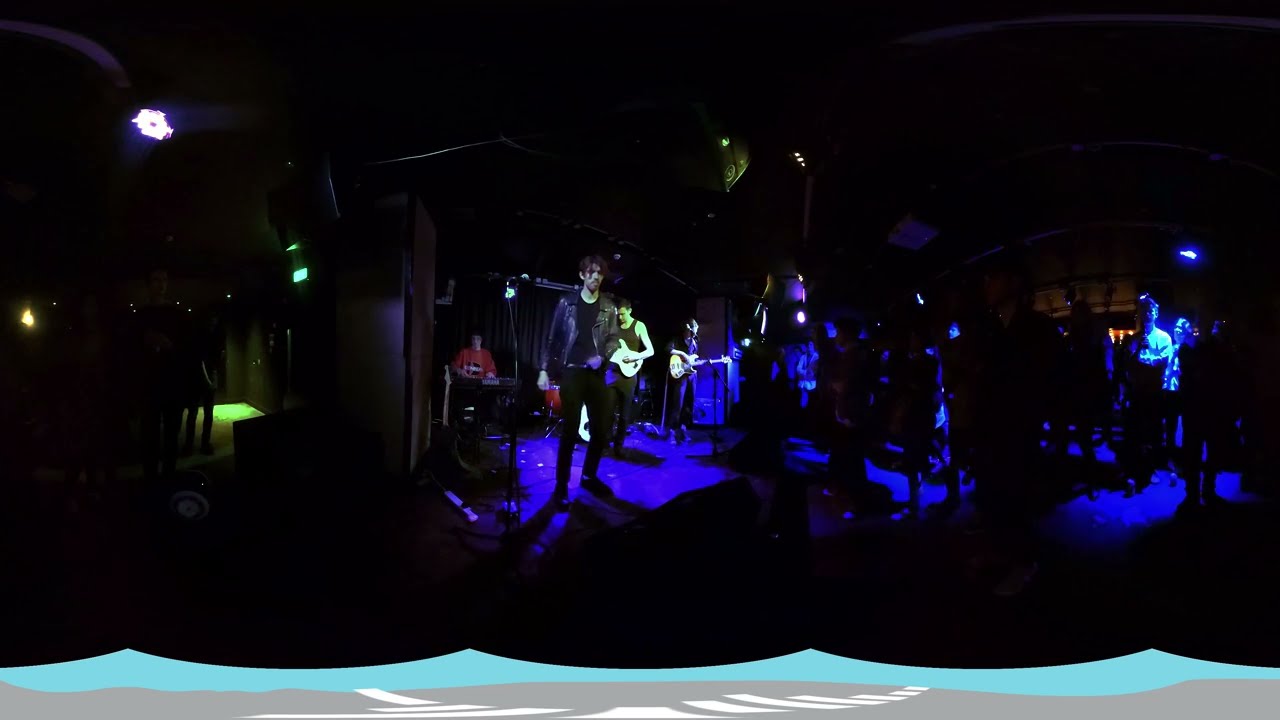The image depicts a dimly lit, indoor stage, presumably in a bar or concert venue, featuring a live band performance. The stage is predominantly illuminated by fluorescent blue lighting that casts neon shadows on the performers. At the front of the stage, the lead singer, dressed in a black leather jacket and black pants, stands at a microphone, appearing to actively engage with the audience. Just behind him stand two guitarists, both clad in black shirts and pants. At the back of the stage, to the right, is a keyboard player wearing a distinctive red t-shirt with a graphic or black emblem on the front. The entire scene is enveloped in a dark ambiance, heightened by the blue lighting and accented by bright white and blue lights visible at the top and middle right of the image. The bottom of the image features a water wave-like graphic, contributing to its unique appearance. The right-hand side of the image seems to show part of the audience, though they are mostly obscured by the darkness and lighting effects.